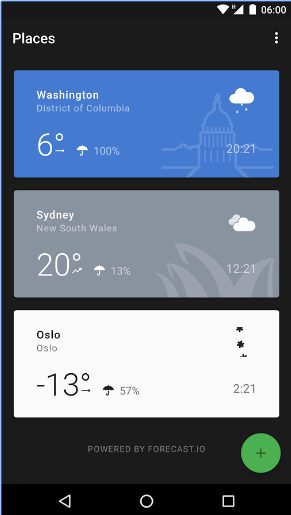**Descriptive Caption:**

The screenshot captures a smartphone display, providing a detailed weather overview for multiple locations. 

**Status Indicators and Time (Top Bezel):**
- The top bezel is black, featuring three key icons on the right: a full Wi-Fi signal, full mobile service bars, and a fully charged battery. 
- The current time is displayed in white, set to military time as "0600."

**Main Weather Section:**
1. **Washington, District of Columbia:**
   - Background: Dark blue.
   - Visual: A light gray or white silhouette of Capitol Hill underneath a rain cloud, with white raindrops.
   - Time: Displayed as "2021" in military format.
   - Location: "Washington" in bold white, followed by "District of Columbia" in regular white text.
   - Temperature: "6°" with an arrow pointing right, possibly indicating Celsius.
   - Precipitation: An umbrella icon with "100%," signifying heavy rain.

2. **Sydney, New South Wales:**
   - Background: Dark gray.
   - Visual: Gray plants on the right side, with a gray storm cloud and a white cloud in front of it.
   - Location: "Sydney" in muted white, followed by "New South Wales" in gray.
   - Temperature: "20°" with an ascending squiggly arrow.
   - Precipitation: An umbrella icon with "13%," indicating a minimal chance of rain.
   - Time: Displayed as "1221," possibly in military format.

3. **Oslo, Norway:**
   - Background: Off-white.
   - Visual: Black snowflakes falling.
   - Location: "Oslo, Oslo" in muted white on the top left, repeated in gray underneath.
   - Temperature: "−13°" with an arrow pointing right.
   - Precipitation: An umbrella icon with "57%," suggesting moderate chances of precipitation.
   - Time: "2:21 PM" in military time format.

**Footer:**
- Reference: "Powered by forecast.io."
- Additional Icons: At the bottom, a green circle with a black X, and a red cross.
- Navigation Buttons: A white, upside-down triangle, a circle, and a square adorn the bottom bezel. 

This detailed weather information offers a comprehensive glance at the current meteorological conditions in three different cities, demonstrating the wide range of weather scenarios.